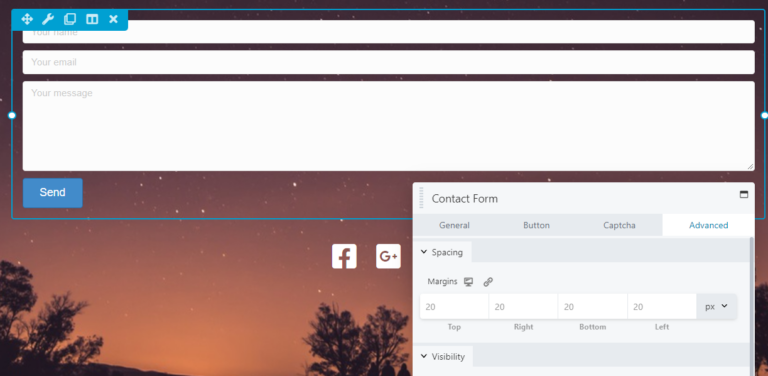This image depicts a user interface of a contact form set against a picturesque background of a twilight sky sprinkled with stars and silhouetted trees. At the top, there are various tool icons available for use. Directly underneath, there are labeled input fields featuring a long white box for the user’s name and another extended white box for the email. Below these fields, there is a spacious text area for the message, providing ample room for detailed communication. Enclosed beneath these fields is a blue "Send" button with blue writing that prompts the action. This section is bordered with a blue line that has two white dots on each end.

On the lower right side of the interface, a pop-up box titled "Contact Form" appears. Within this box, users can access options labeled "General," "Button," "Captcha," and "Advanced," with the "Advanced" tab highlighted in blue. This section also offers spacing adjustment options with margin settings for the top, right, bottom, and left. Additionally, there is a visibility setting contained within a white bar set against a gray background.

In the bottom corners of the image, there are small white squares each containing a Facebook and Google icon, respectively. The entire contact form and tools are superimposed on a beautiful background showing the sky adorned in shades of red and orange mingling with dark tree silhouettes, lending the image a serene yet dynamic appeal.